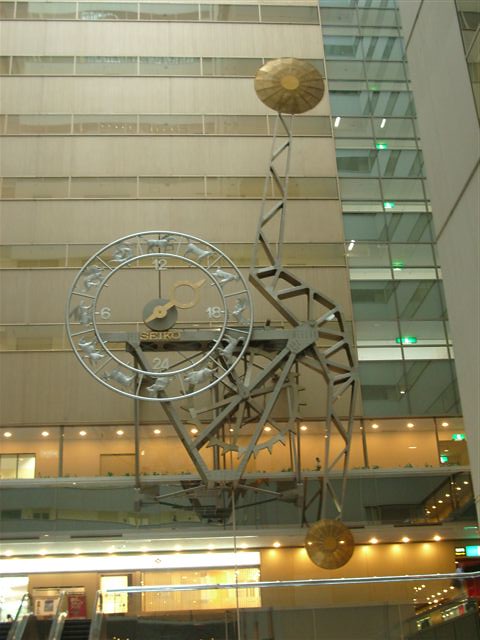The image depicts a multi-story building, possibly a mall or an office complex, featuring numerous floors and large windows that reflect surrounding structures. The building, which is beige, has well-illuminated lower levels, with visible lights on the ceiling, an escalator at the bottom level, and likely elevators. Dominating the center of the image is an intricate metal sculpture, doubling as a clock made by Seiko. This artistic structure includes a large golden plate at the top and a smaller one lower down, with metal components throughout. The clock displays time in an unconventional manner with 12, 18, 24, and 6 positions replacing the traditional numbers, accompanied by animal symbols. Despite its artistic nature, the clock does function, although it's somewhat challenging to read.